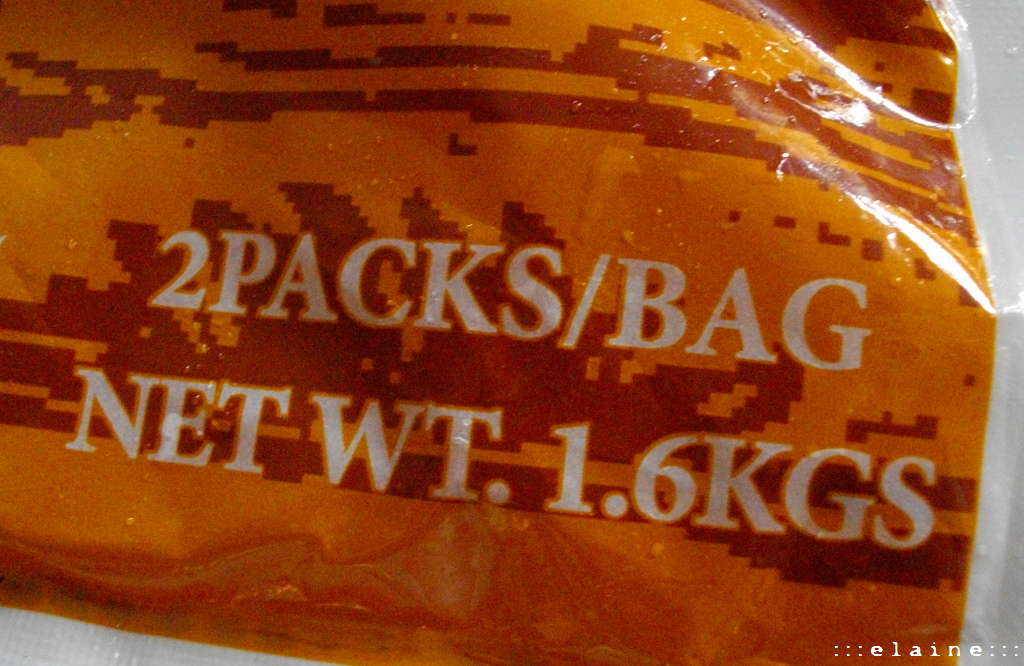The image showcases a close-up view of an orange bag with brown stripes, set against a white background. The rim of the bag is white, creating a striking contrast with the orange and brown hues. The camera focuses on a specific section of the packaging, where the text "Two Pack / Bag" is prominently displayed in bold, white letters. Just below, it reads "Net Weight: 1.6 kgs," also in entirely white typography. 

Given its appearance, the bag resembles those typically found in the freezer section of a grocery store, likely used for packaging frozen foods such as french fries. The bag is slightly crumpled on one side, and the light reflects off its glossy, plastic surface, adding a tactile dimension to the visual.